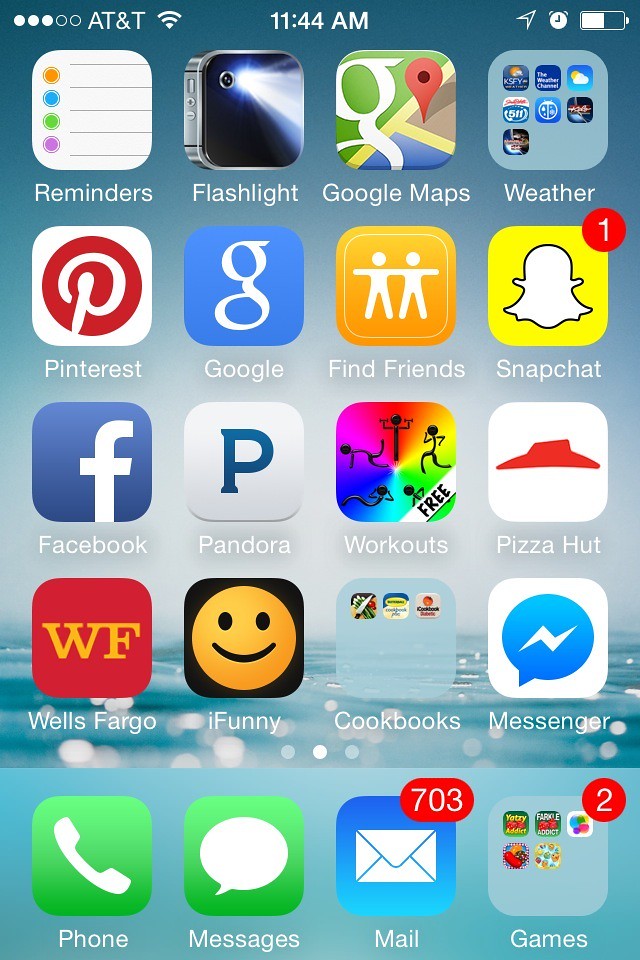A detailed description of an iPhone screen, displaying a variety of apps against a light blue, water-themed background. The screen shows numerous icons, including Phone, Messages, Pinterest, a notebook app, Snapchat, Find Friends, Google, Pandora, Facebook, Pizza Hut, a workout exercise app, Wells Fargo, iFunny, and a cookbooks app. The cookbooks app contains three sub-icons. Additionally, there's a Messenger app, a Mail app with 703 unread messages, and a folder containing five different game icons with two notification badges. Other notable apps include Google Maps, a flashlight tool, a weather app with seven sub-apps, and Snapchat with one unread notification. The device is connected to AT&T network, shows a Wi-Fi signal at three out of five bars, and indicates the time as 11:44 AM. The battery is approximately 50% charged.